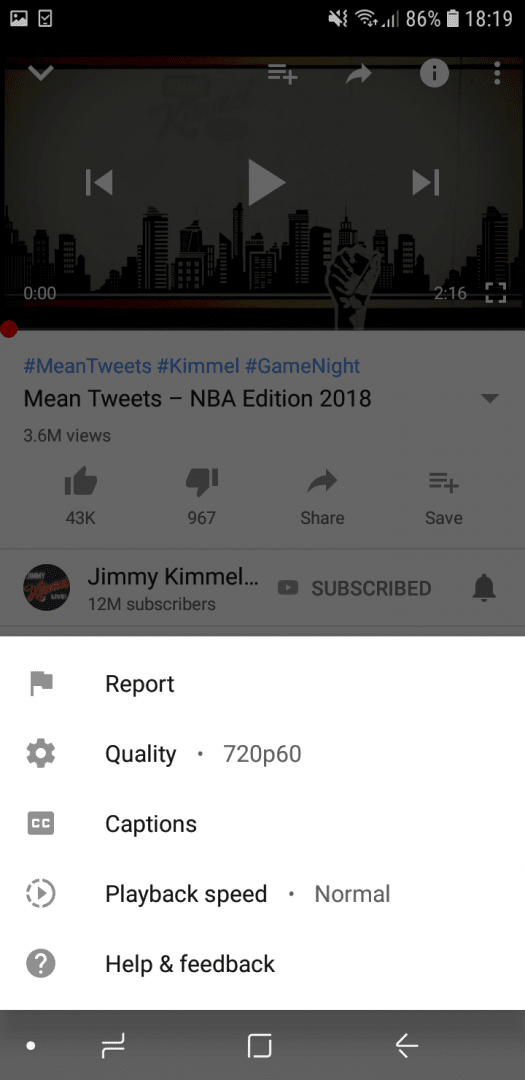The image is a screenshot of a website displayed on a cell phone. At the top of the screen, there is a black banner. Within this banner, there is an icon of a white square with the outline of a mountain inside it. Next to this, there is another square icon with a black background and a white check mark. Moving rightward, there are symbols indicating the phone’s status: a volume icon with a diagonal line through it, followed by WiFi and cellular signal icons, the battery level at 86%, and the time displayed as 18:19 (6:19 PM).

Below this banner is another section that appears to have an overcast shadow effect, possibly due to a pop-up at the bottom. The background shows an image of a cityscape. Superimposed on this are media control buttons: a play button, a rewind button, and a fast-forward button. Beneath these controls, text reads "Mean Tweets NBA Edition 2018." There are interactive icons for thumbs up, thumbs down, sharing, and saving the content. The text shows the name “Jimmy Kimmel” and notes that he has 12.12 million subscribers.

Toward the bottom of the screen, a white pop-up banner is visible with options including "Report," "Quality," "Captions," and "Playback Speed" set to "Normal." There are also options for "Help" and "Feedback." At the very bottom, another black banner is present.